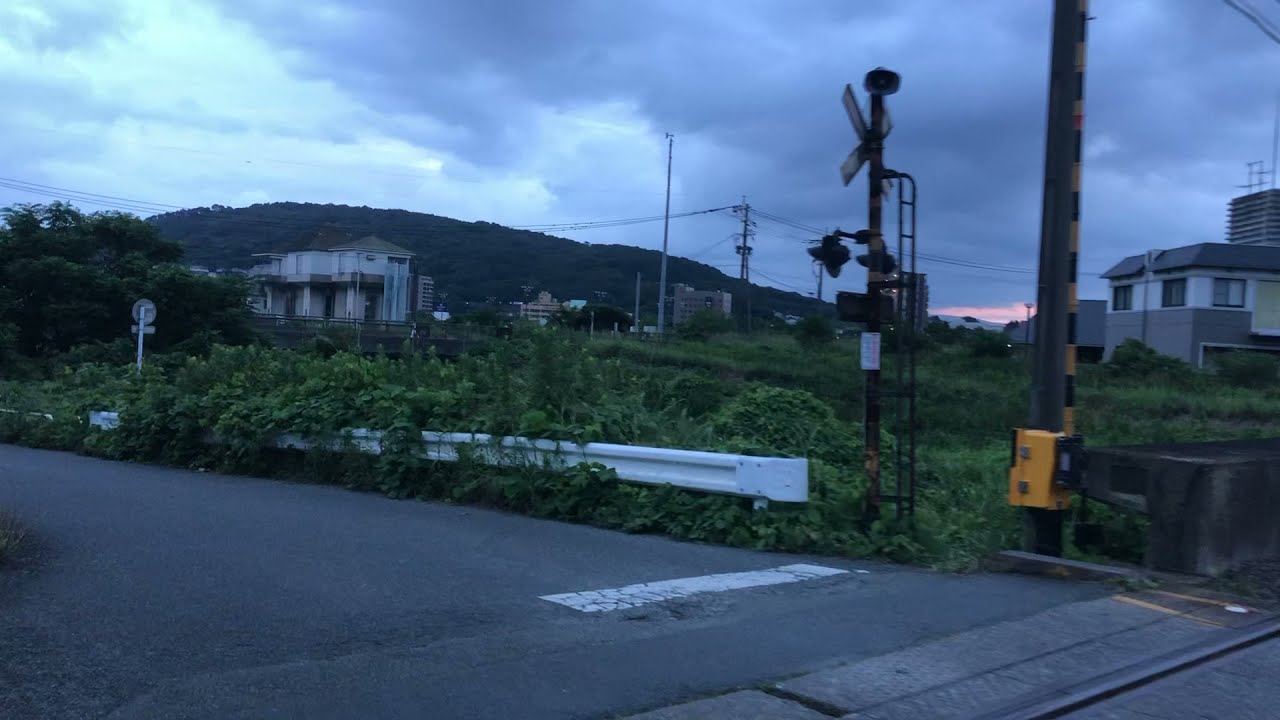This wide, rectangular daytime photograph captures a scenic intersection of a paved road and a railroad track in a residential area with an industrial touch. The road, bordered by a white metal railing intertwined with lush green bushes, starts from the bottom left and stretches towards the bottom right corner. At the road’s intersection with the train tracks, there are distinct black and yellow railroad crossing arms and the characteristic X sign. The landscape is dotted with wooden utility poles and streetlights, their power lines stretching across the scene. In the foreground, dense brush and weeds thrive, while multiple signs add to the urban feel. The backdrop features multi-story buildings, including what appear to be Asian-style houses, along with industrial structures. Majestic mountains loom in the distance under a sky laden with gray and white clouds, with a hint of sunlight breaking through, creating a serene yet dynamic atmosphere.